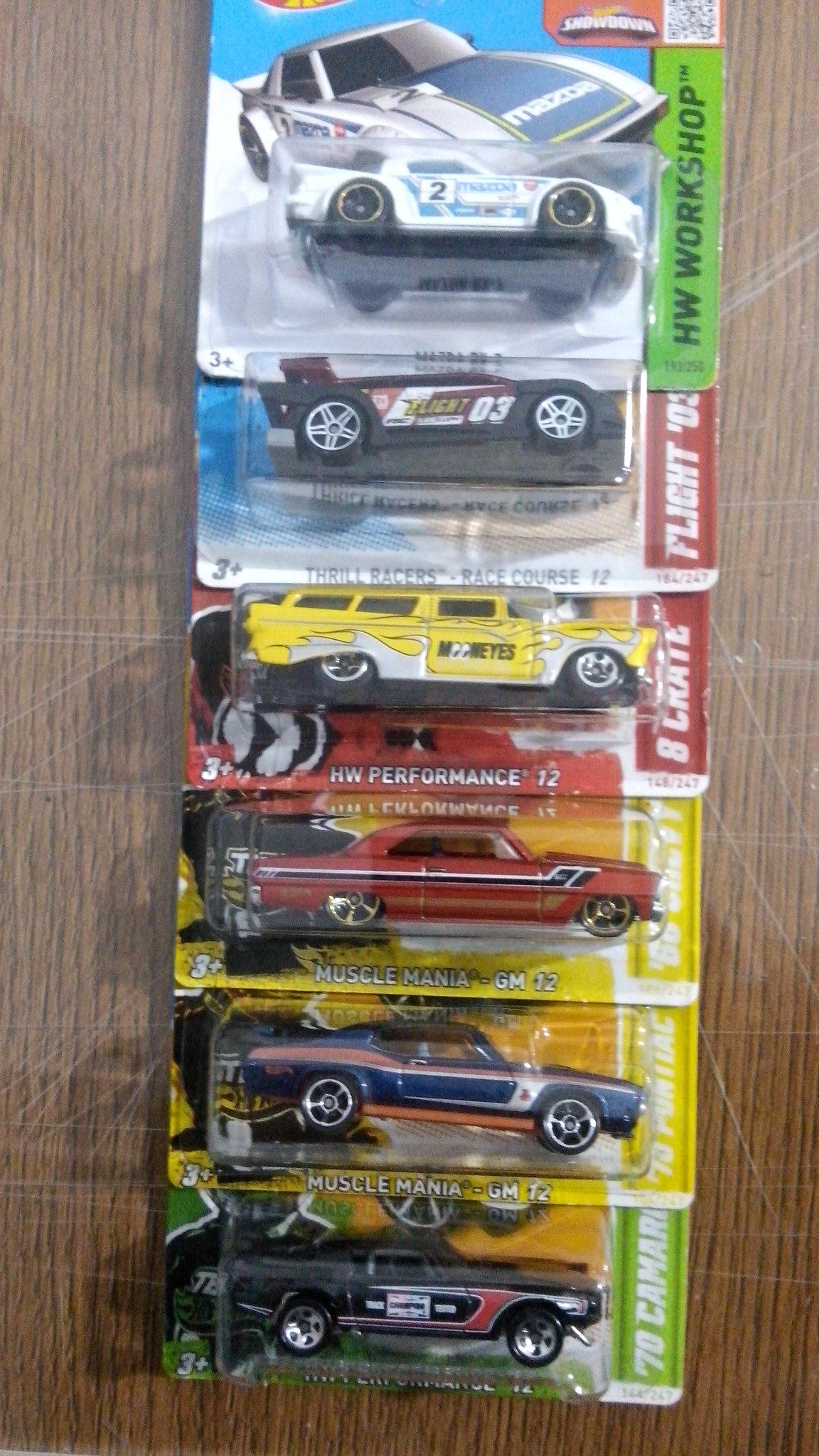The image captures a vertical, color snapshot of six Hot Wheels cars still in their retail packaging, meticulously arranged in a stacked formation on a scratched wooden surface. Each car is encased in a plastic bubble attached to a colorful cardboard backing, showcasing vibrant hues of green, yellow, red, and blue. From top to bottom, the cars include: a white car with blue designs, a maroon car with white designs labeled with “number three,” a yellow vehicle adorned with white flames and the text "Moon Eyes" and "Hot Wheel Performance 12," a red sports car with a white and black horizontal line marked "Muscle Mania GM12," and a blue car featuring an orange and white line. Each package indicates "3+" suitable age, with some featuring texts like "Muscle Mania" and "Thrill Racers," all illuminated under bright lighting with sharp shadows, highlighting their colorful, vintage race car aesthetics.